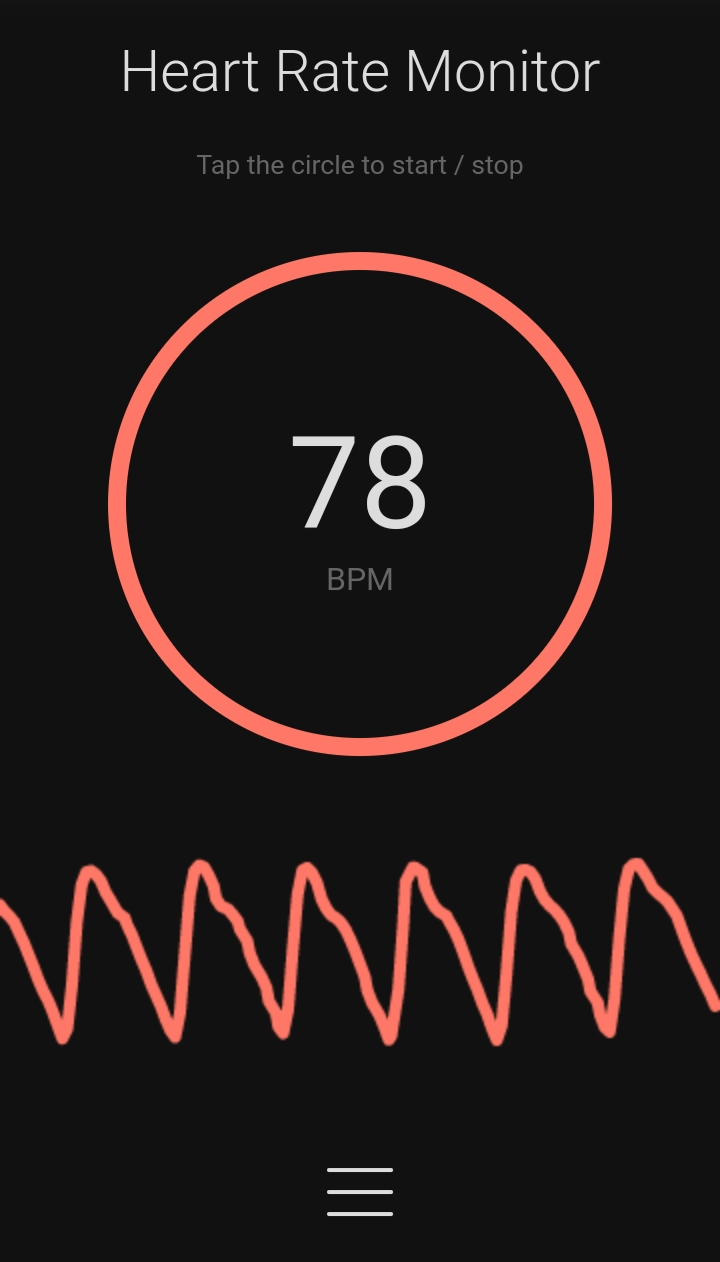The image appears to be a screen grab from a health monitoring app displayed on a smartwatch or other device. The background is completely black. At the top, in white lettering, it states "heart rate monitor." Just below that, in smaller white text, it reads "tap the circle to start/stop." Centrally positioned, there is a large circle outlined in red. Inside the circle, the number "78" is displayed in white, indicating the current heart rate, with "BPM" (beats per minute) written just below it in smaller white text. Below the red circle is a fluctuating red line signifying the heart rate pattern. At the bottom of the image, three horizontal white lines are stacked, suggesting a menu option.